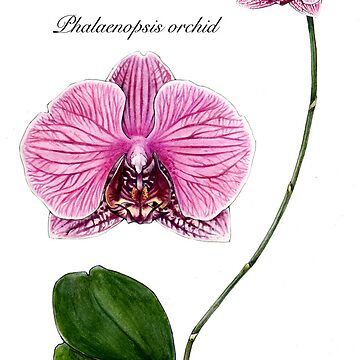The image features a stylized digital drawing of the Valenio Fis Orchid. In the upper left corner, the title "Valenio Fis Orchid" is prominently displayed. Below the title, a detailed depiction of an orchid flower petal is shown, viewed straight on to highlight its intricate veined areas and the distinctive face-like structure found within the petal. To the right of the flower petal, extending vertically from top to bottom, is a large leaf with a stem that appears to connect to the flower petal. The stem is long and detailed, and attached to it are two leaves. The colors in the image include various shades of pink, purple, white, green, brown, and black. The overall style suggests an educational or artistic context, perhaps something one might see in a classroom setting, focusing on plant anatomy and botanical illustration.